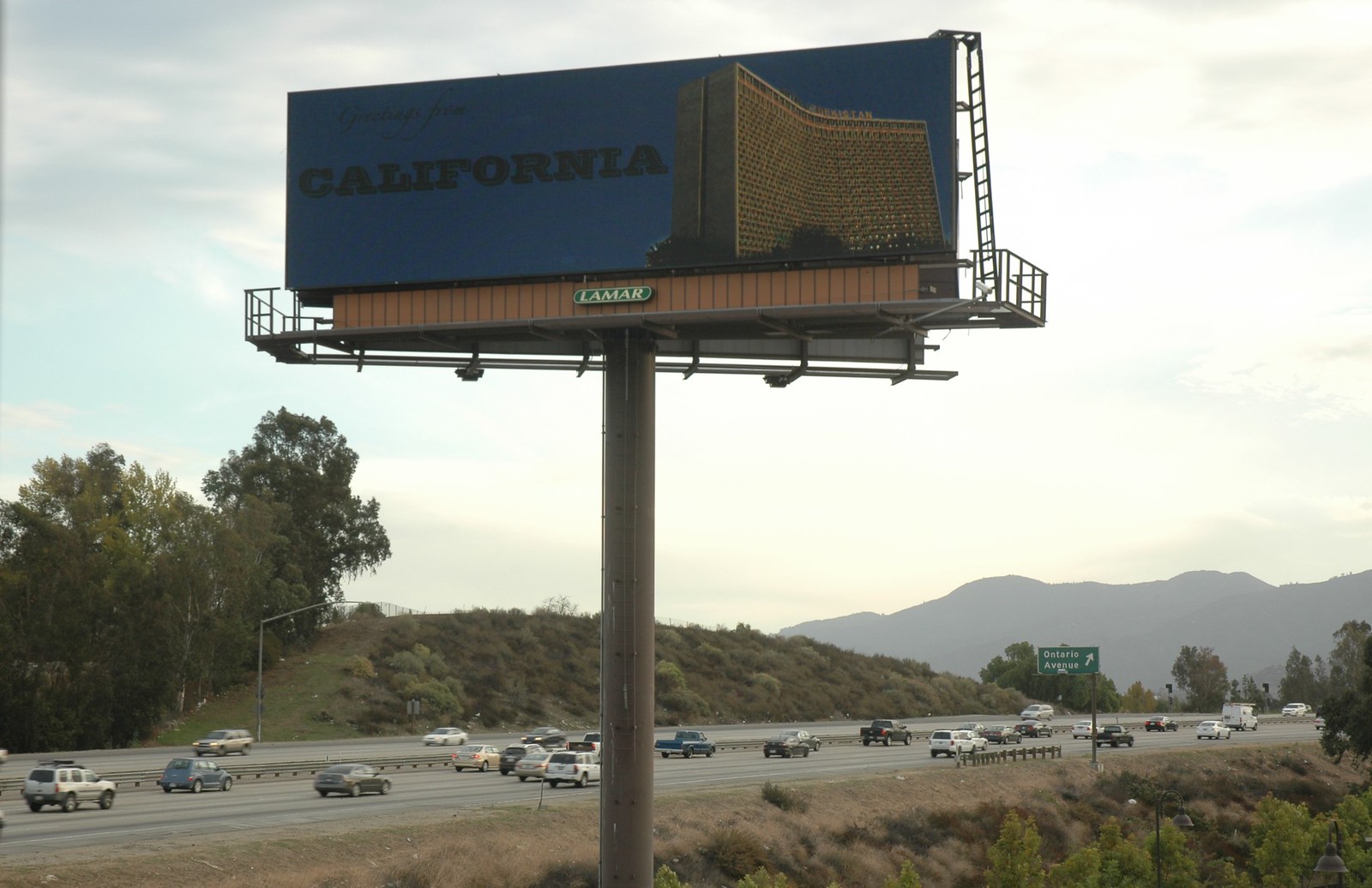A bustling highway stretches out towards a distant mountain ridge, with traffic moving in both directions under a hazy, light sky. In the foreground, the highway features three lanes heading away from the viewer, brimming with various cars. On the other side, an equal number of lanes accommodate fewer vehicles moving in the opposite direction. A prominent road sign indicates an upcoming ramp, though the details on the sign are indiscernible. Dominating the scene is a towering billboard sponsored by Lamar, mounted on a substantial metal pole with accessible stairs. The billboard, which faces both sides of the highway, prominently advertises a grand hotel named "The California," potentially hinting at a destination or the allure of the state itself. The backdrop features a mountain range or ridge, faintly visible through the atmospheric haze. The sky above is a muted white, adding to the overall serene tone of the image.